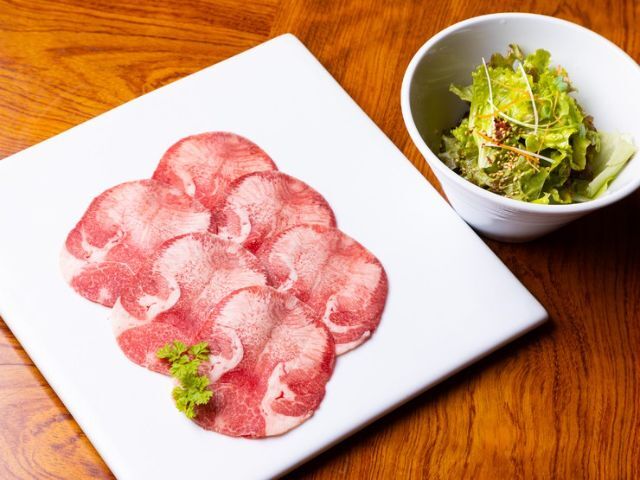This photo, taken indoors, captures a top-down view of a food setting presented on a medium brown wooden table with visible grain. The focal point is a modern, square white plate displaying six slices of pinkish-red meat, possibly uncooked and marbled with fat. The slices are arranged in two neat layers of three, with a delicate sprig of pale green parsley adding a touch of aesthetic appeal. To the upper right of the plate is a small white bowl containing a salad with chartreuse-colored leaves, sprinkled with an undetermined seasoning and a few long, white slices that resemble cheese. There are no utensils visible, enhancing the minimalistic and possibly Asian-inspired presentation of the dish.